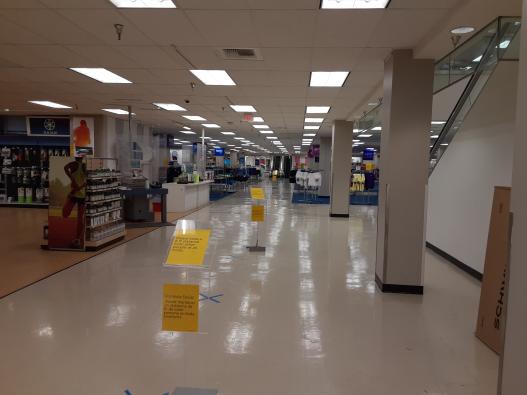The photograph captures the interior of a high-end department store, reminiscent of a Macy's or J.C. Penney. Dominating the right-hand side is a triangle-shaped sidewall formed by the black railing of an upward-moving escalator. Progressing along the right side from near the camera into the distance is a series of tan pillars with black bases. The off-white ceiling features a series of 8-10 square recessed fluorescent lights, casting a reflection onto the glossy white floor tiles below. Centrally located on the floor are multiple yellow signs, though the text is illegible. Initially, two of these signs are visible near the bottom of the image, with two more placed further down the aisle.

On the left side of the image, there are displays that appear to be dedicated to cosmetics or lotions, organized for easy browsing by shoppers walking down the wide, white-tiled aisle. An indistinct alcove, possibly for shoes or socks, is also visible on the left. In the far distance, the image shows a multitude of clothing racks, both straight and cylindrical, adorned with garments in white and darker colors. Additionally, the left side hints at a sporting goods section, marked by an image of a person running and presumed sports-related merchandise on display.

The ceiling also houses vents and sprinkler systems amidst large, continuous white panels of fluorescent lighting. The distant view of the store reveals assorted sections and items of various colors, including some indistinct blue items, contributing to the impression of a sprawling retail space divided into numerous departments, some carpeted and some bare-floor.